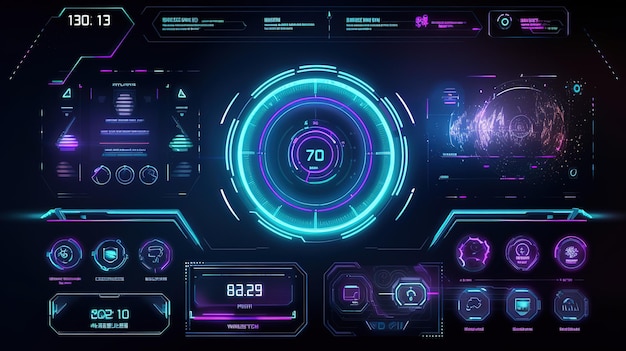The image depicts a highly modern car dashboard, dominated by a sleek, black background with various controls and displays illuminated in vibrant shades of fluorescent blue, light blues, dark blues, and lavender. Centrally located is a prominent speedometer with two concentric circles; the outer ring is in blue, encircling a smaller purple circle that displays the number "70" in blue digits.

To the right of the speedometer, there is a rectangular display area featuring an image of a circle or a globe. In the upper left corner of the dashboard, "130:13" is printed in white. Below this, five small sections of text are visible, with the first three in blue and the last two in a pinkish-purple, though the exact content is unreadable. 

Additional buttons and controls are scattered across the dashboard; they appear on the left and right sides, as well as in the lower sections of the image, though their labels are too small to decipher. On the lower left, within a beveled rectangular area, "202:10" is printed in blue, adjacent to another white print reading "82.29."

The image, rectangular in shape and approximately four inches wide by two inches high, showcases an array of advanced technological features, suggesting a vehicle cockpit rich with functionality and modern design.